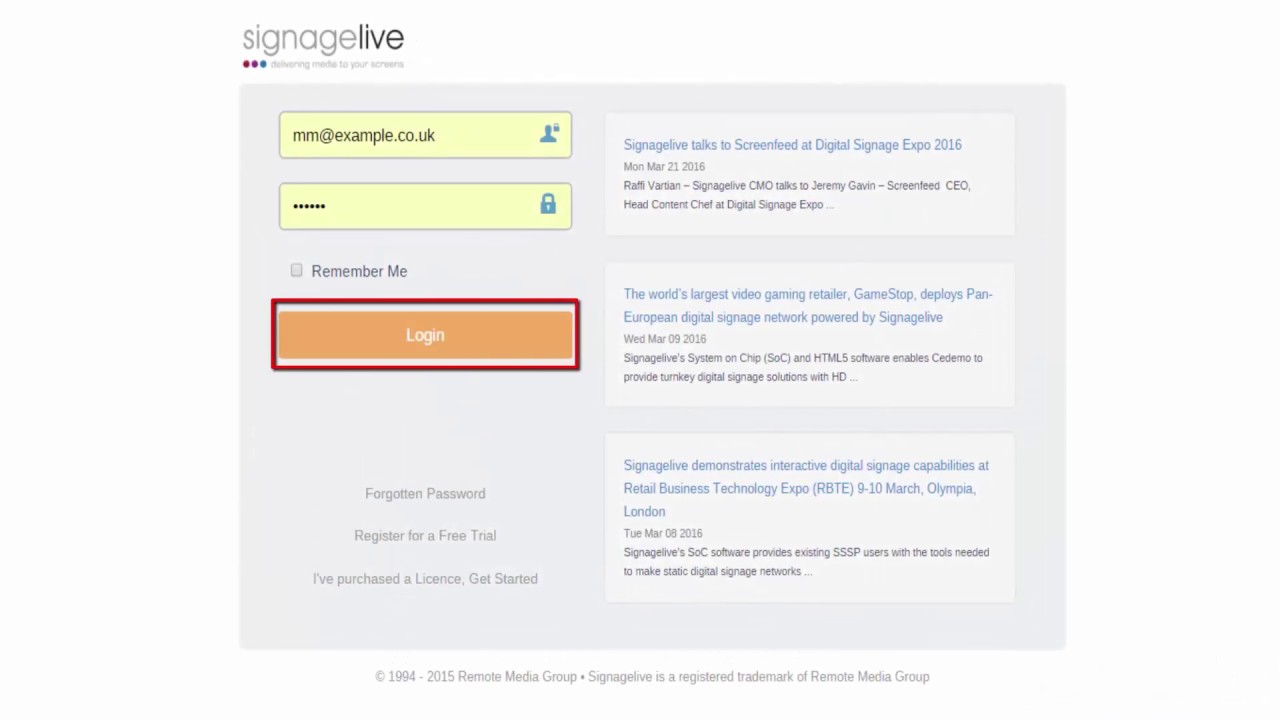**Caption:**

This screenshot showcases the Signage Live login page, encapsulated within a large gray box. The primary elements include two yellow fields for user credentials: one for the email address (example.co.uk) and another for the password. Below these fields is an orange login button outlined in red. Additional navigational options include "For me," "Register for free trial," "I purchased a license," and "Let's get started."

To the right of the login section, news highlights from Signage Live are displayed. These include:

- **March 21, 2016**: An interview at the Digital Signage Expo 2016 where Signage Live CMO Rafi Viratan speaks with Jeremy Gavin, CEO and Head Content Chief of ScreenFeed.
- **March 9, 2016**: Announcement of GameStop deploying a pan-European digital signage network powered by Signage Live.
- **March 8-10, 2016**: Demonstration of interactive digital signage capabilities at the Retail Business Technology Expo in Olympia, London, featuring Signage Live’s System on Chip (SOC) and HTML5 software solutions for existing SSP users.

The detailed overview emphasizes Signage Live's involvement and advancements in the digital signage industry, highlighting interviews, deployments, and technological demonstrations.